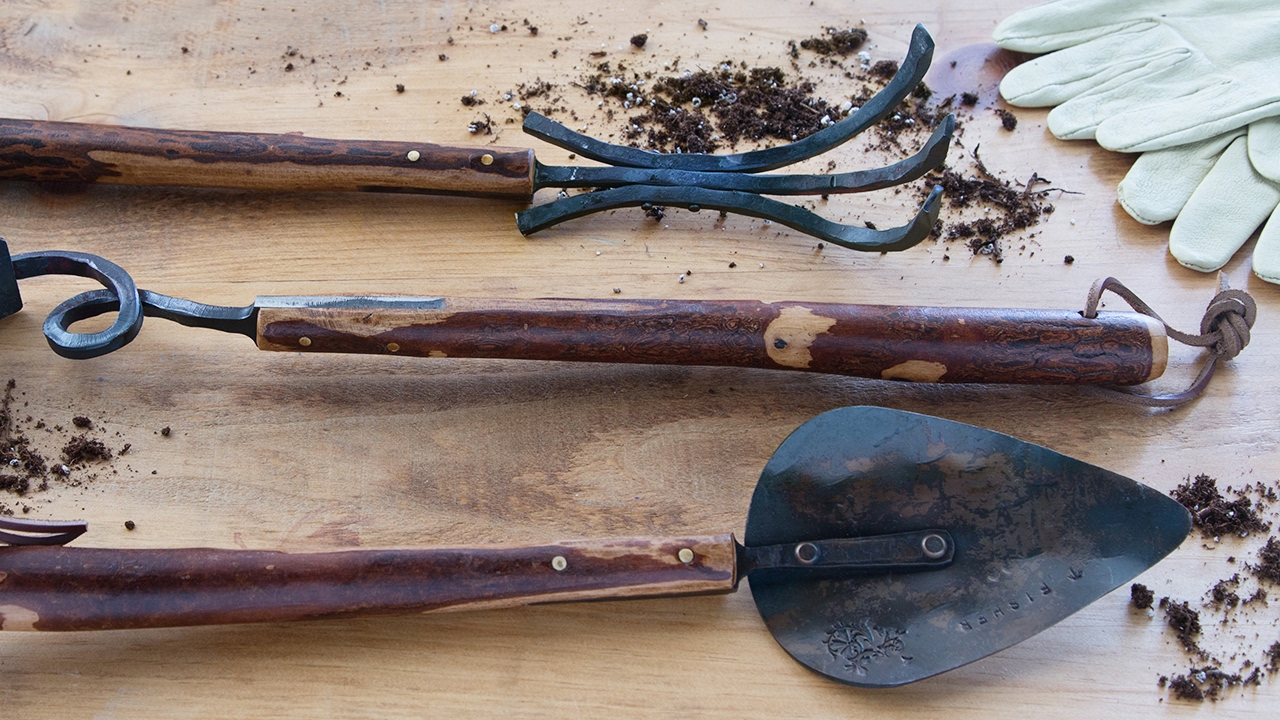This photograph captures a trio of vintage gardening tools and fragments of white gardening gloves, artfully arranged on a light wooden surface scattered with bits of dirt. At the top of the image is a hand rake, featuring three curved, wrought iron hooks designed for raking soil. In the middle lies an enigmatic tool with a knotted leather strip at the handle's end, its working part obscured from view, but the handle displays a twisty corkscrew design. The bottom tool is a hand trowel, resembling the shape of a guitar pick, crafted from hammered wrought iron. Each tool features long, hand-carved wooden handles. The tools are oriented horizontally with two facing right and one facing left, evoking a sense of casual placement rather than a professional arrangement. The white gardening gloves, partly visible in the top right corner, add a touch of practicality to this nostalgic, earthy ensemble.